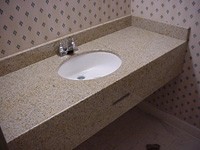In this small, square image captured within a bathroom setting, a long rectangular sink is prominently featured, mounted against the wall in a corner. The sink, white and recessed into its base, boasts a sleek silver faucet and a matching silver drain at its center. Above the sink, the wall is adorned with decorative wallpaper, showcasing a pattern of dark, diamond-like shapes against a white background. The base of the wall is trimmed with wide molding that appears to be made of plastic or wood, adding a touch of elegance to the space. The light-colored tile flooring enhances the room's brightness, which is softly illuminated by ample lighting.